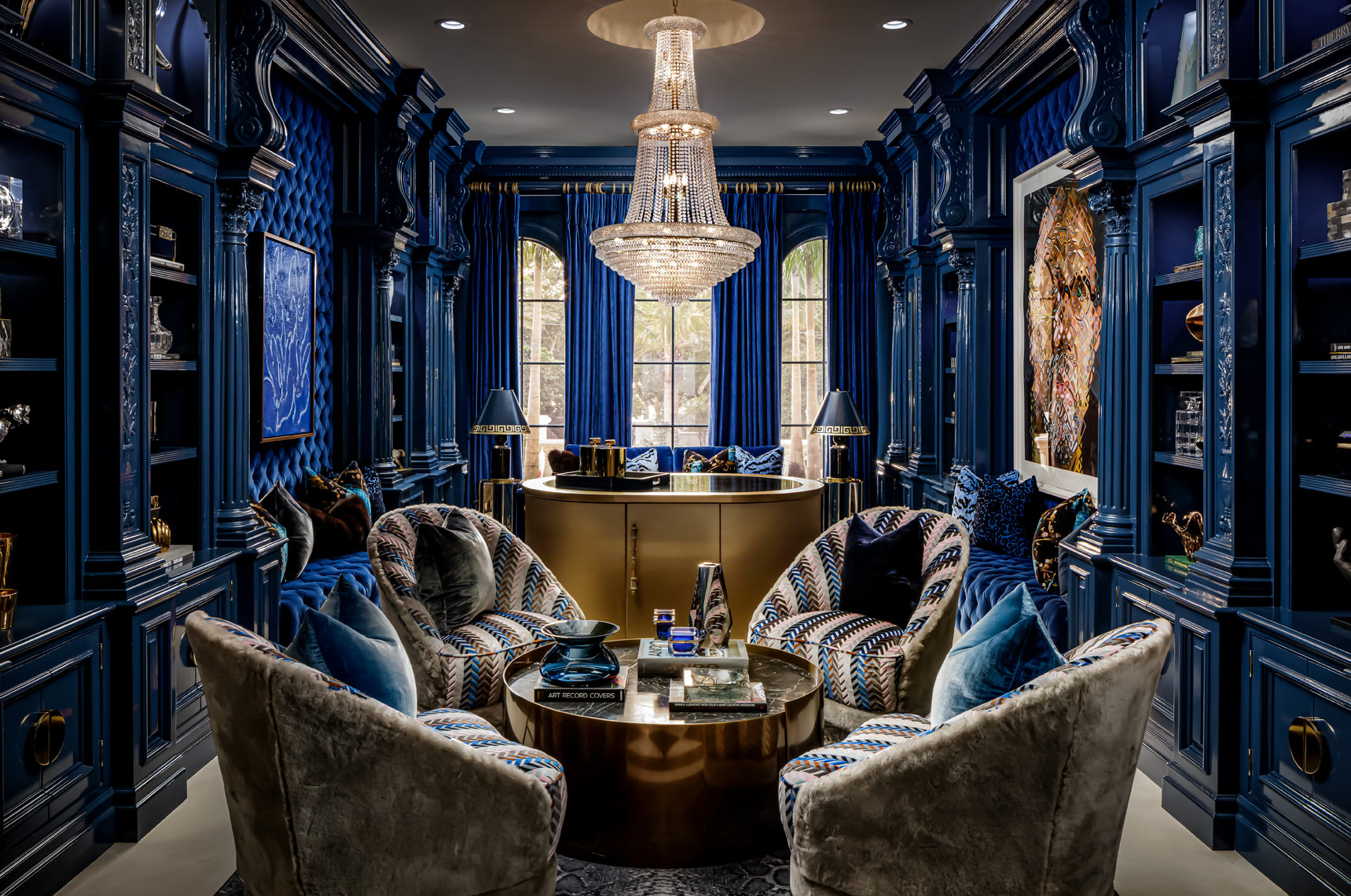The image depicts an intricate and luxurious room with an elaborate blue theme and white accents. The walls are painted a medium shade of blue, matching the four panels of floor-to-ceiling curtains that frame three tall windows in the background. Between the windows, the walls feature padded, tufted sections adorned with pieces of artwork. Large, built-in bookcases, also in medium blue, occupy the side walls, adding to the room's sophisticated ambiance.

In the middle of the room hangs a grand, white crystal chandelier, which illuminates the space with a soft glow. Beneath the chandelier, arranged in a circular formation, are four plush chairs upholstered in a tan, blue, and brown fabric, each accompanied by a pillow in varying shades—two light blue, one black, and one tan. At the center of this seating arrangement stands an ornate, metallic gold table. Resting on the table are several objects including books, a blue vase, and possibly a black tray with indistinguishable items or canisters. 

The ceiling is painted white and features skylights that enhance the room's natural lighting. On one of the side walls, there's a picture of a man's face, contributing to the room's refined decor. The overall design, with its luxurious elements and meticulous attention to detail, creates an atmosphere of opulence and comfort.